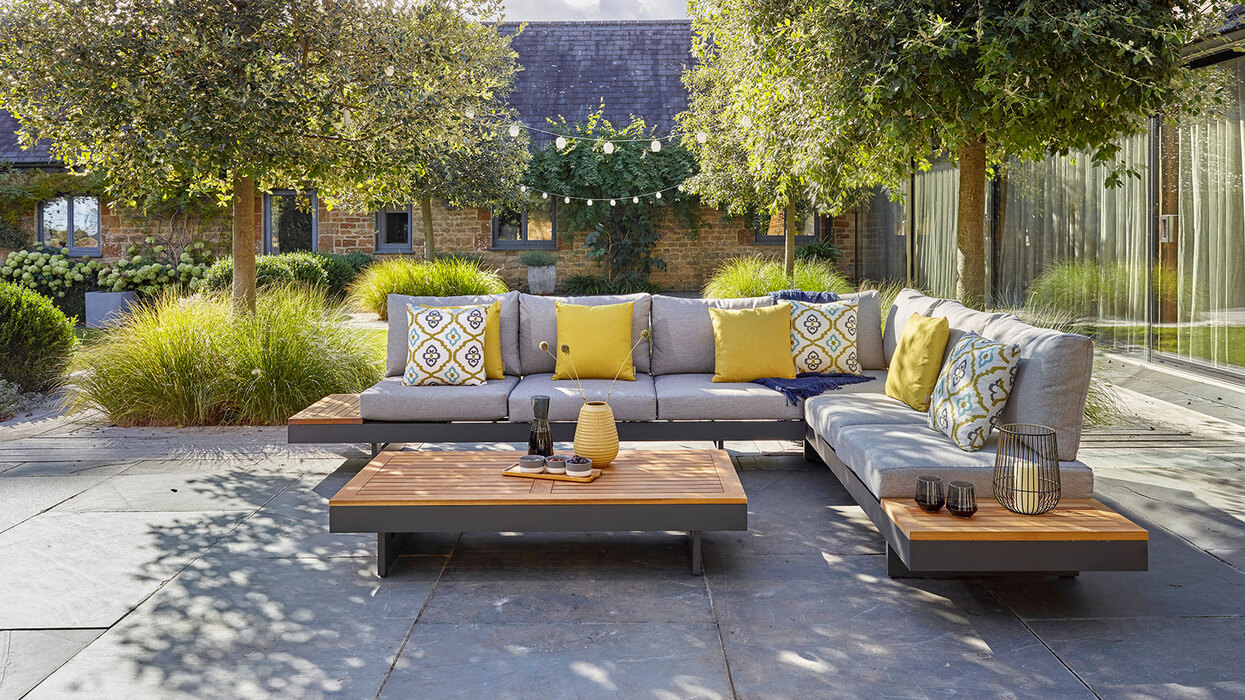This photograph captures a sunny day in a courtyard, possibly of a hotel or apartment building, featuring an outdoor patio setting. The focal point is a gray sectional sofa, arranged in an L-shape with square cushions. Each end of the sectional features a wooden platform that doubles as a side table. The nearest platform holds a large candle enclosed in a wire candle holder and two small cups. The sectional is decorated with an assortment of pillows: a blue and gold patterned one, several yellow ones, and another blue and gold pillow at the corner where a blue blanket is draped over the far cushion.

In front of the sofa sits a wooden-topped coffee table with a steel-colored base. On this table rests a dark vase, another vase filled with dried weeds tipped with yellow, and three candle holders. To the left of the sofa is a tree with tall grass planted at its base, accompanied by tufts of tall grass and a couple of bushes behind it. 

The patio is surrounded by a glass-fronted building with long white curtains. The sun casts clear shadows across the slate-tiled ground. Further in the background, there's a brick building with a slate-gray roof and gray door and window frames. Overhead, strings of lanterns add a decorative touch to the setting, completing the inviting outdoor ambiance.